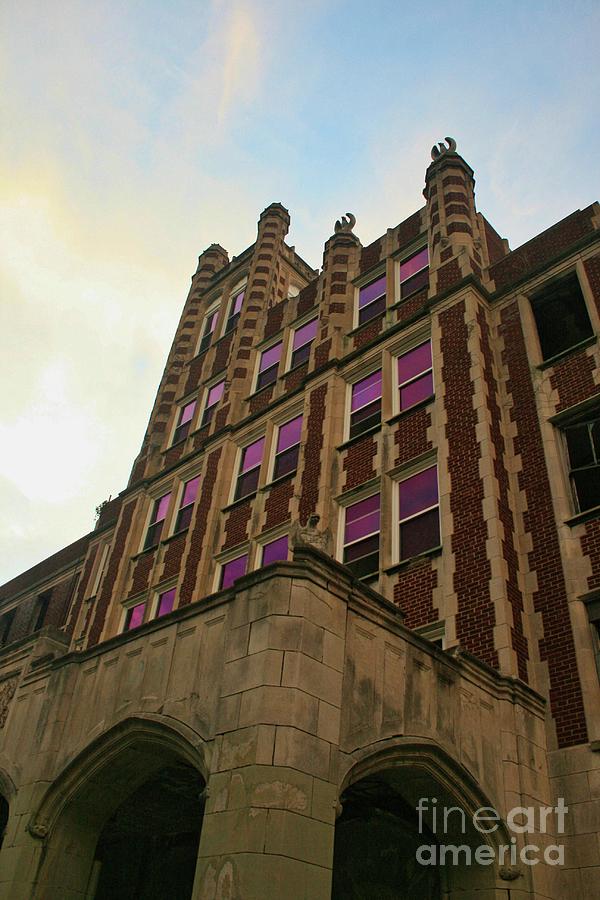This photograph captures the upward view of a majestic, castle-like brick building adorned with white and beige accents, taken from ground level. The structure features a prominent overhang entryway about 8 to 15 feet above the ground, with two large arched openings in the stone base, resembling passageways for vehicles. The architectural details include staggered dark and light brown block patterns at the corners and between rooms, giving it a vintage aesthetic. Rising five stories high, each window is fitted with a pink window shade at the top, and many have a distinctive purple shine possibly reflecting a distant sunset or digitally enhanced. At the pinnacle of the building, faint outlines of gargoyle-like figurines stand against a bright, white sky. The bottom right corner of the image features the logo "Fine Art America" in white lettering, suggesting the photograph is trademarked by the art service.